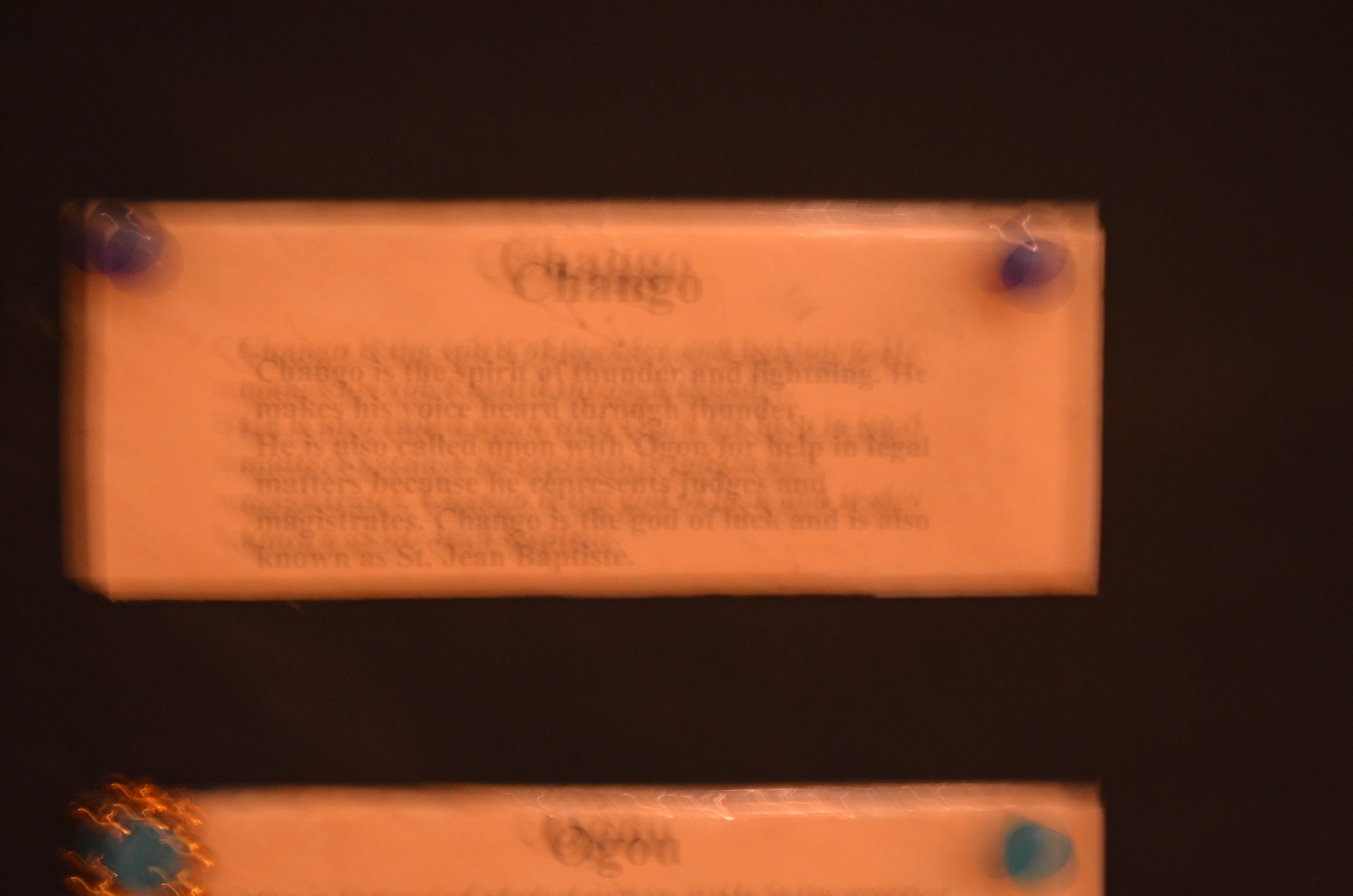This photograph is a very blurry close-up taken against a black background. It prominently features two pink rectangular pieces of paper or plaques, each appearing to be tacked onto a surface. The tacks are distinctly colored, with the first paper held by purple tacks and the second by turquoise tacks.

The first plaque, though difficult to read due to the blurriness, has the word "Chango" printed in bold black letters at the top. Beneath "Chango," there is additional text in black print, but it’s mostly illegible due to the double vision effect in the photograph. From what can be deciphered, Chango is described as the spirit of thunder and lightning, known for making his voice heard through thunder. He is invoked alongside Ogon for assistance in legal matters, as he symbolizes judges and magistrates. Chango is also recognized as the god of luck and is associated with Saint Jean Baptiste.

The second plaque, lower in the image and also blurry, bears the name "Ogon" at the top but lacks further discernible details.

The composition and details, though blurred, suggest an attempt to relay the significance of these spiritual figures and their cultural relevance.